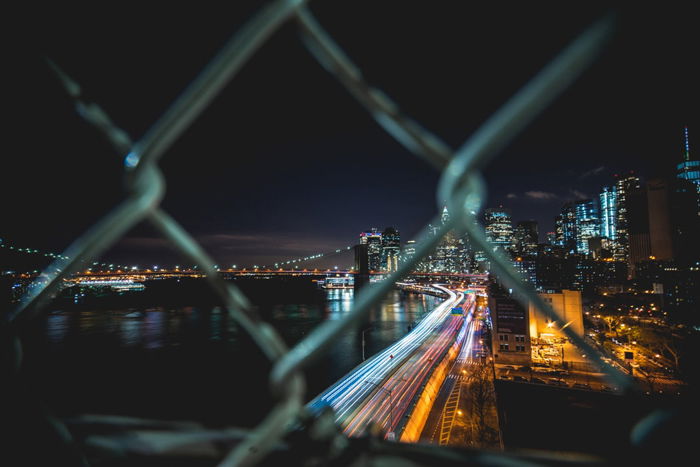Captured at night, this professionally-taken cityscape is viewed through a blurred chain link fence, its X-shaped links clearly visible in the foreground. The photograph was taken from a high vantage point, likely a bridge, and features a sprawling, horizontally-oriented panorama. To the right, a cluster of tall buildings, their illuminated windows glowing brightly against the dark sky, stretches vertically. A curved road, bustling with traffic captured in slow shutter speed, creates streaks of yellow and blue light as it winds to the left towards a river or riverfront. In the distance, a suspension bridge with cables soaring upwards stands prominently, hinting at the depth of the cityscape. The scene is a vibrant juxtaposition of darkness and light, with the freeway's blurry lights and the twinkling city lights reflecting off the water, painting a dynamic and lively urban portrait.